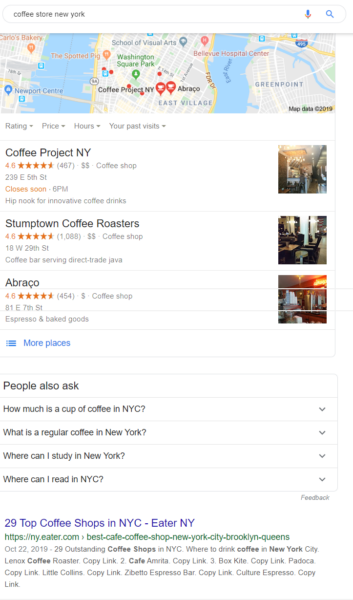In the image, we have a screenshot of a Google search results page for the query "coffee store, New York." At the top, there's a Google search bar displaying the search term. To the right of the search term, there is a voice-to-text microphone icon, followed by a blue magnifying glass icon for initiating the search.

Directly below the search bar, filling about 20% of the total height of the image, there is a map highlighting several pinned locations representing coffee stores in New York. Below the map, the top three suggested results are listed.

1. **Coffee Project New York**:
   - Star Rating: 4.6 stars
   - Address: Listed below the rating
   - Hours of operation: Provided beneath the address
   - Thumbnail Image: Present on the right side

2. **Stumptown Coffee Roasters**:
   - Star Rating: 4.6 stars
   - Address: Listed below the rating
   - Hours of operation: Provided beneath the address
   - Thumbnail Image: Present on the right side

3. **Abraco**:
   - Star Rating: 4.6 stars
   - Address: Listed below the rating
   - Thumbnail Image: Present on the right side

Below these listings, a blue text link indicates "More places." Further down, black text signifies a section titled "People also ask," featuring four collapsible drop-down boxes with popular queries. The first two visible questions are: "How much is a cup of coffee in New York City?" and "What is a regular coffee in New York?"